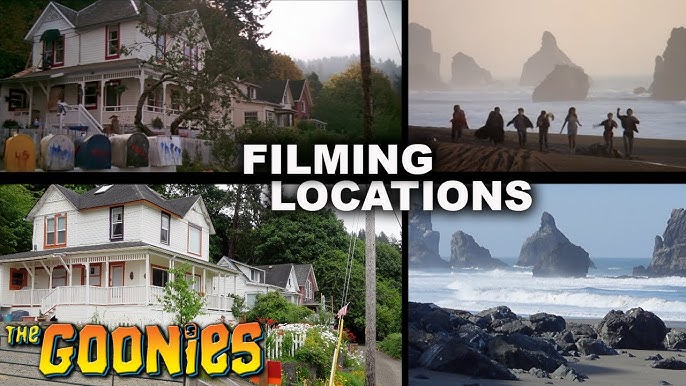A detailed and coherent caption for the image, using details from each voice description, would be:

The image is a composite of four photographs divided into quadrants, showing "The Goonies" filming locations. In the center, in white text, it reads "filming locations," with "The Goonies" in distinctive green text in the larger lower-left quadrant. The top-left and bottom-left images feature a two-story American house with a tattered appearance in the past, including several worn mailboxes, contrasted with a more recent, tidy version of the house, devoid of the unkempt mailboxes and showcasing a well-maintained yard. The top-right and bottom-right images depict a beach scene; the top-right photo shows a group of seven kids running on a foggy, rocky beach, reminiscent of a scene from the movie, while the bottom-right image presents the same beach clearer and free of people, highlighting the specific filming location's transformation over time.